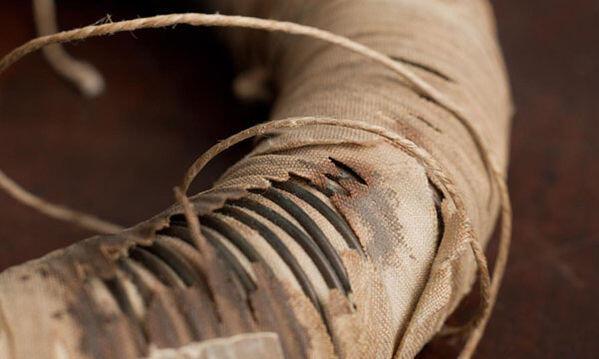The photograph depicts a mysterious object that is difficult to definitively identify. The main subject of the image is an arm-like or pipe-like form, wrapped in a tattered, light brown fabric that resembles a bandage. This cloth, frayed and torn in places, reveals underlying black wires or rubber bands coiled around the object, giving the appearance of shoe laces. Additionally, light tan ropes or twine encircle the object in two loops, contributing to the rough, makeshift appearance. The object is set against a blurred, dark brown backdrop that may include elements such as a red and black tiled floor and possibly a chair leg in the upper left corner, adding to the enigmatic nature of the scene. The overall effect suggests age and damage, with areas of darker discoloration hinting at burn marks or stains on the fabric wrapping.